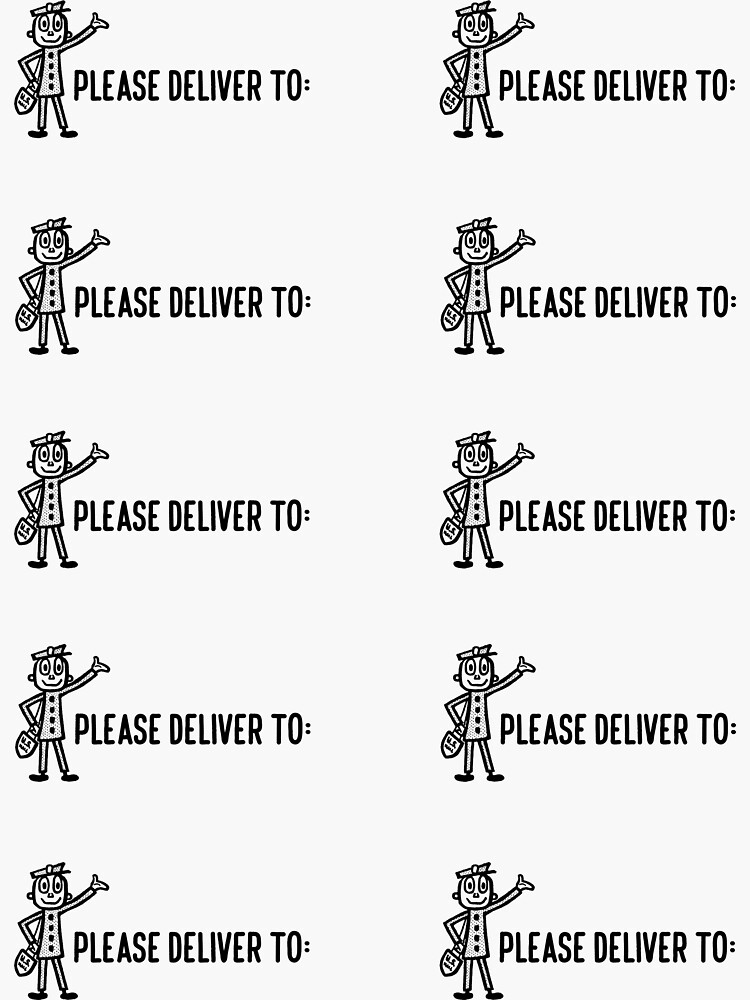The image consists of a sheet of white paper featuring multiple prints of the same label design, repeated ten times in a grid format. Each label showcases a simplistic, almost stick figure illustration of a postman. The postman is depicted with one hand raised in the air and the other resting on his hip, with a mailbag slung over his shoulder bearing the text "US MAIL." The illustration includes rudimentary details such as buttons down the front of his shirt, a circle for a head with a big smiley face, two large eyes, and an old-fashioned mailman's hat. Adjacent to the postman, the text "PLEASE DELIVER TO:" is written in bold, all-capital letters. This design is arranged in two columns of five labels each, occupying the left and right sides of the paper.